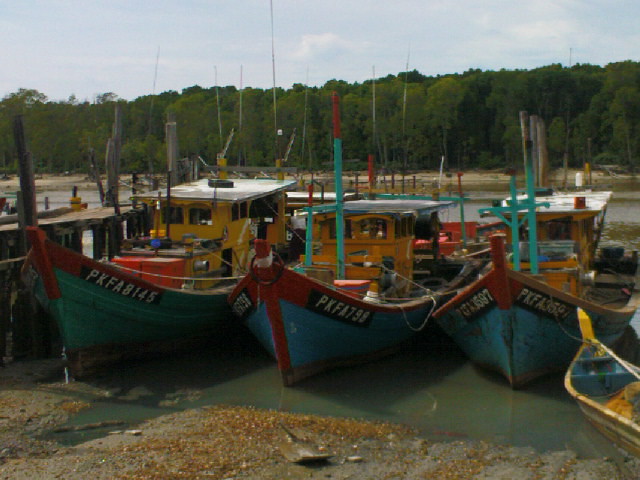This detailed photograph showcases three sizable wooden fishing boats docked at a sandy, tree-lined shoreline. Each boat has a distinctive color scheme: two boats feature blue hulls with red trim, while the leftmost boat has a green hull accented with burgundy red. All the boats display registration numbers starting with "PKFA" followed by additional digits, prominently painted in white on black stripes along their sides. At the front of each boat, there are arched windows, and flat metal roofs cover yellow cabins that resemble small houses.

Distinctive teal poles, one tipped in red, are mounted on the vessels. On the deck of the leftmost boat, there are visible red boxes. The water around the boats appears shallow, a murky greenish-gray, suggesting low tide or perhaps infrequent use. Partially visible in the bottom left corner is the tip of a yellow and blue rowboat or canoe, adding a touch of diversity to the scene. The backdrop includes a densely wooded area with a sandy and muddy beach, scattered with downed logs and debris. This setting collectively exudes a sense of quiet abandonment and rustic maritime charm.